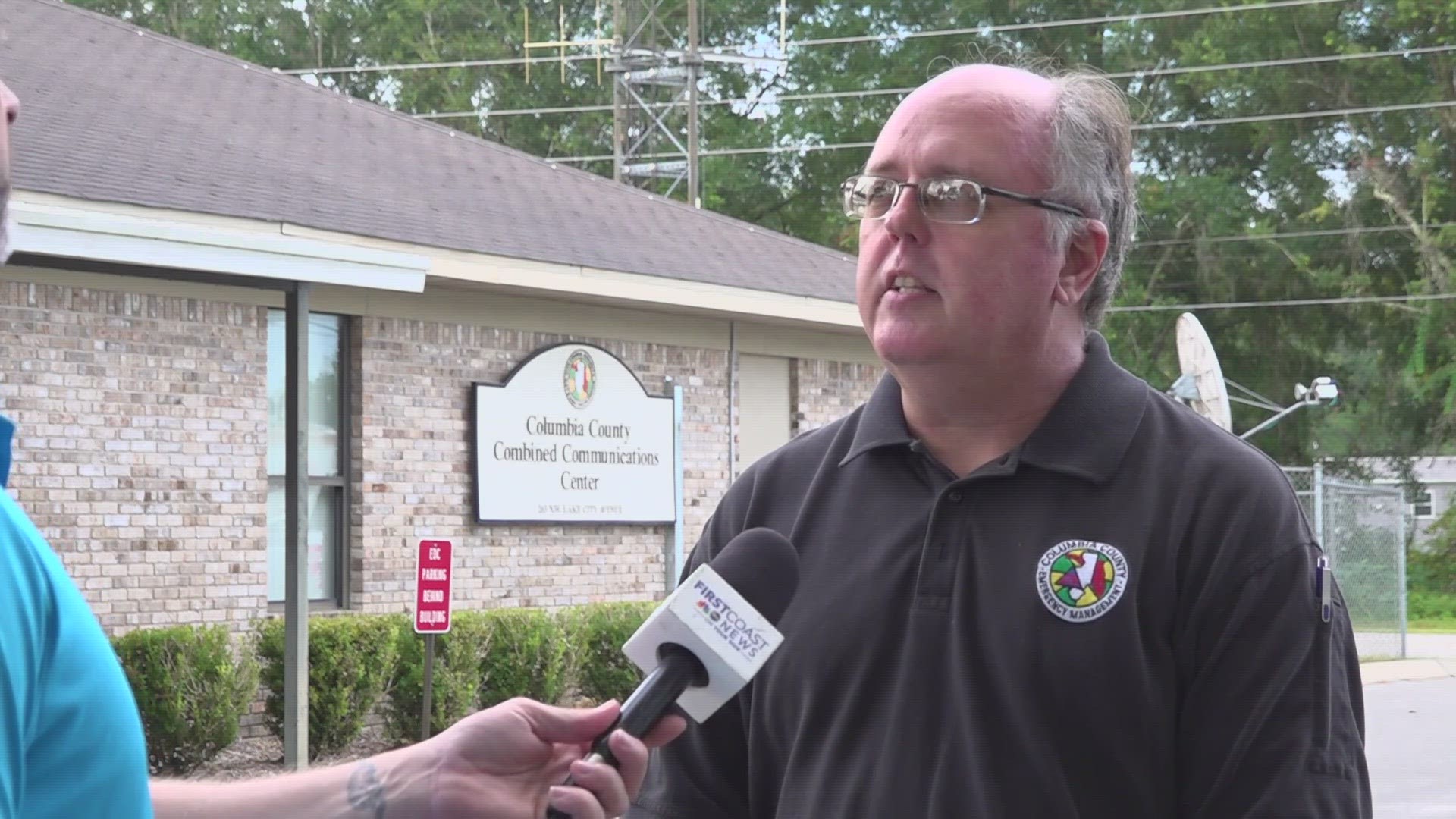The image depicts an older man, possibly in his late 50s or 60s, who is moderately overweight and partially bald with graying brown hair. He is wearing glasses with clear rims and a brown polo shirt that features a logo on the left side of his chest, matching the logo on the building behind him. He is being interviewed outside the Columbia County Combined Communication Center, a one-story brick building. The man interviewing him is only partially visible, showing just a shoulder and arm, which appears to be in a turquoise short-sleeved shirt. The interviewer holds a black microphone with a white box that likely bears a station logo. Visible in the background are elements of the communication infrastructure, such as satellite dishes and antennas, along with what appears to be a parking lot.